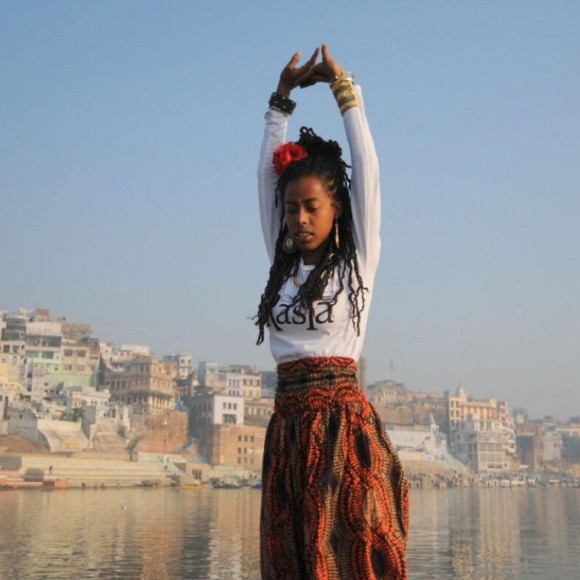This photograph depicts a young Black woman, likely in her 20s, standing outdoors in the immediate foreground. She has long cornrowed hair pulled back, cascading over her chest and adorned with a red flower. Her arms are raised above her head, fingers interlocked, as if she is stretching or practicing yoga. Her eyes are closed, exuding a serene expression. She is dressed in a long-sleeved white shirt with black text partially obscured by her hair; it seems to read "RASTA" or "RASJA." She wears golden bracelets on her wrists and dons a detailed, ornate skirt with intricate brown designs, appearing embroidered or beaded, along with a beaded girdle around her waist. 

In the background, a body of water stretches out behind her, leading to a Mediterranean-style coastal town situated on a sloping hillside. The town features multi-story rectangular buildings in various shades of red, light brown, and white brick or stone, terraced one above the other, creating a dense urban landscape. The sky above the hillside is a pale blue, suggesting a midday or late afternoon setting.